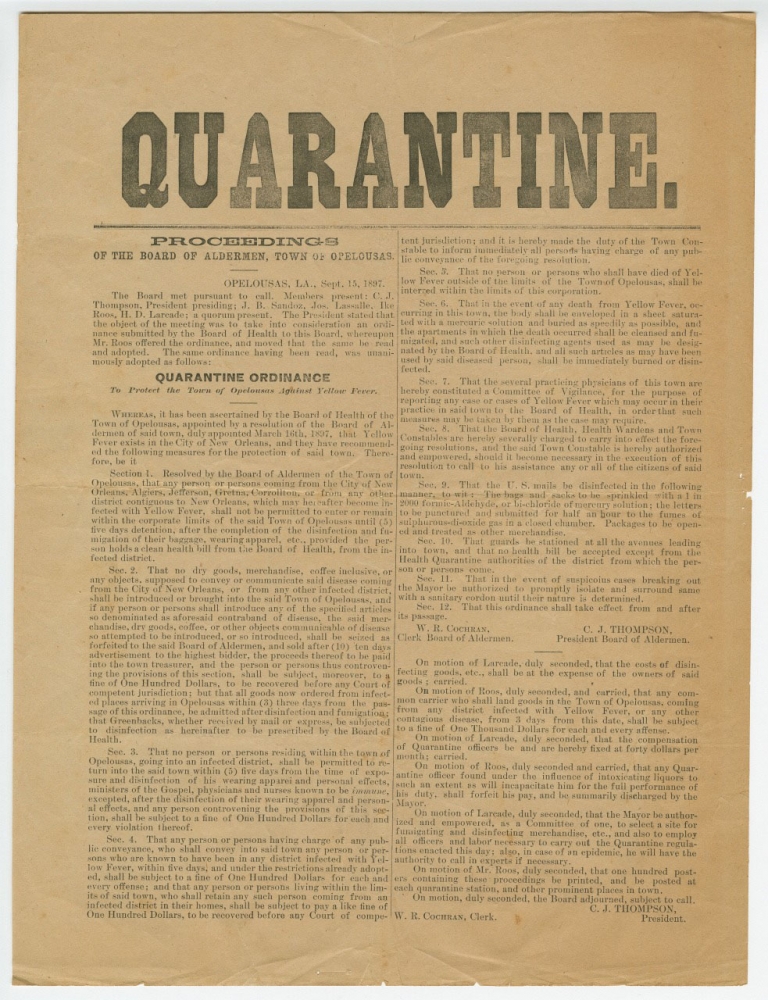This image is a photograph of an old, tan-colored newspaper or magazine page, with the letters printed in a faded black ink. The page is worn and looks quite historic, resembling old notices similar to those seen in Western movies. The heading, in large, bold, blocky capital letters, prominently reads, "QUARANTINE." A period follows this heading, beneath which there is a smaller, but clearly printed, title stating, "Proceedings of the Board of Aldermen, Town of Opelousas," dated September 15, 1897. The text underneath is faint and small, comprising two full columns that detail the proceedings and include the "Quarantine Ordinance" aimed at protecting the town from yellow fever. The ordinance specifies sections 1 through 12, outlining the various rules and restrictions. The document is signed by C.J. Thompson, President of the Board of Aldermen, and mentions other members present at the meeting, including J.B. Sandoz and Joe Lassall. The ordinance states that the quarantine measures were recommended by the Board of Health to mitigate the spread of yellow fever from New Orleans, detailing the constraints and precautions the town must adhere to during the quarantine period.